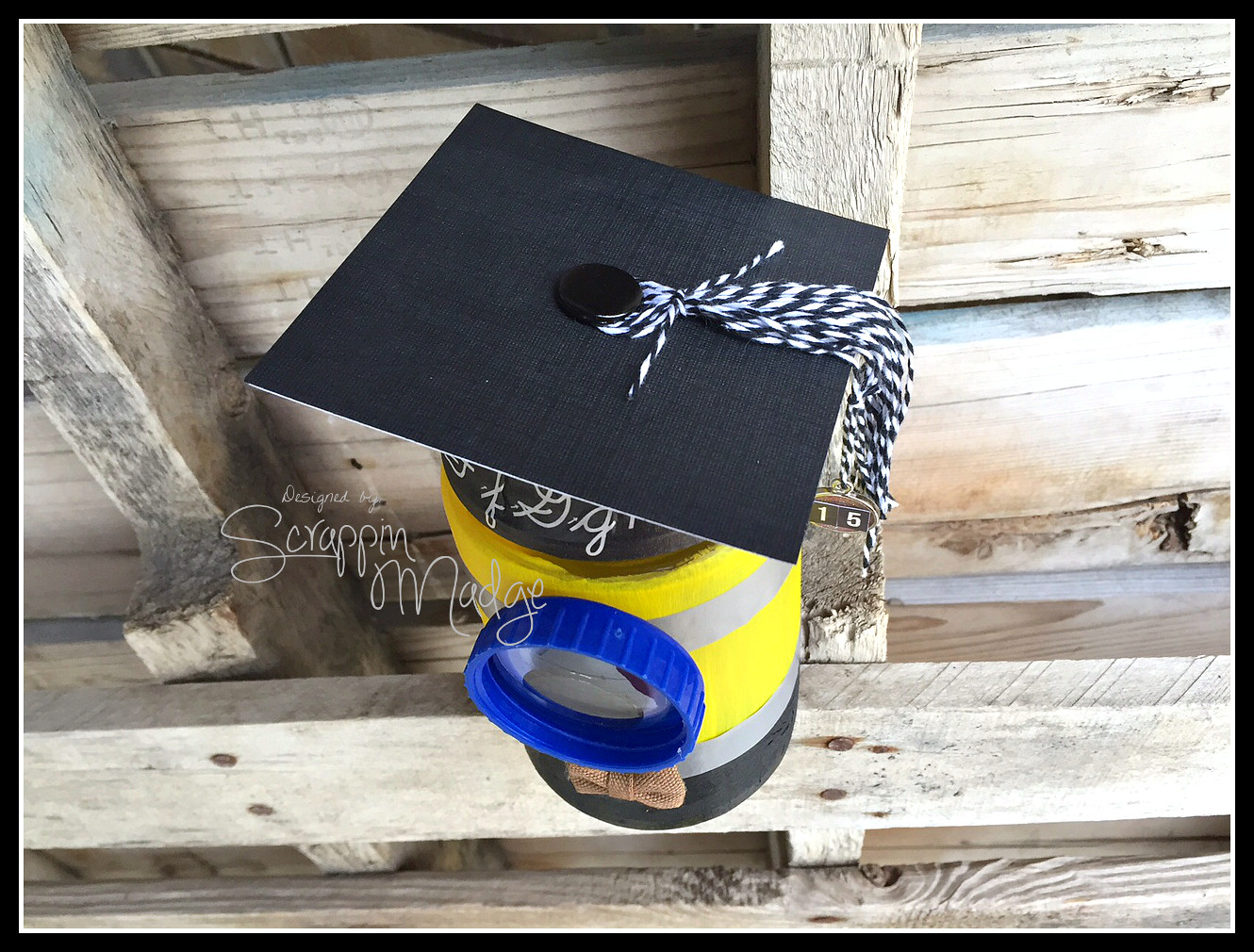The photograph depicts a whimsical creation designed to resemble a graduation-themed minion character from the popular movie franchise. The structure appears to be a crafted totem or statue made from a series of cylinders and jars, featuring a black base cylinder transitioning into alternating yellow and gray stripes, capped with a blue lid intended to mimic an eyeball. Beneath the "eye," a brown bowtie is affixed, enhancing the minion-like appearance. Crowning this playful figure is a black graduation cap adorned with a black and white tassel, anchored by a red button at its center. This cap also has a note with illegible text on its side. 

The creation is set against a rustic wooden backdrop composed of planks secured by rusty flathead nails, adding a homecrafted, vintage charm to the scene. Overlaying the image is elegant script reading "designed by Scrapp & Madge," a testament to its handcrafted nature. The overall impression is a detailed and thoughtful portrayal aimed at capturing the essence of a graduating minion, complete with a celebratory graduation cap and playful detailing.